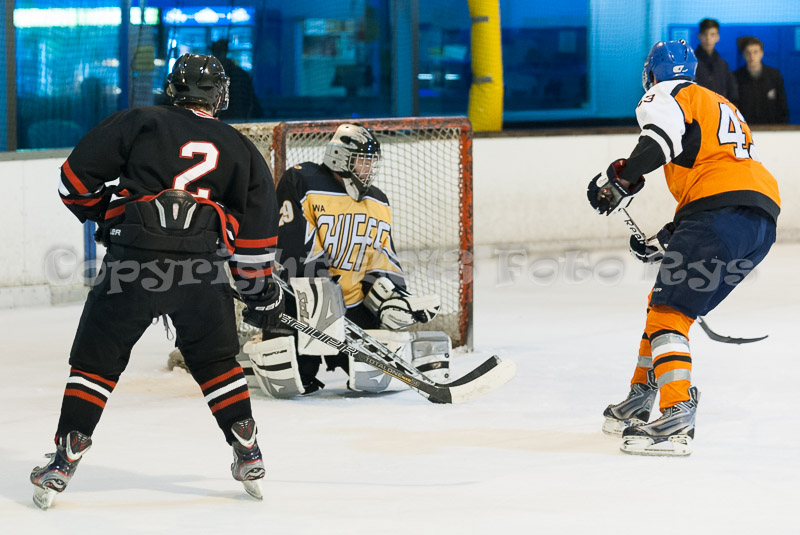The image depicts an intense moment in an ice hockey game, clearly marked with a watermark stating "copyright photo RYS." At the center of the scene, a goalie in a yellow, black, and white jersey, bearing the word "CHEAPS," is kneeling in a blocking stance in front of a goal framed with orange metal and white netting. He is surrounded by two opposing players, each wearing distinctly different uniforms. One player, clad in an orange and blue jersey with matching navy blue shorts and orange socks, is positioned on the right, skating determinedly toward the goal. Another player, dressed in a red, white, and black jersey, faces toward the goal from the left. In the background, the rink is illuminated with blue lighting, and two bystanders can be seen observing the match from outside the rink’s boundary, adding to the scene's dynamic and immersive atmosphere.